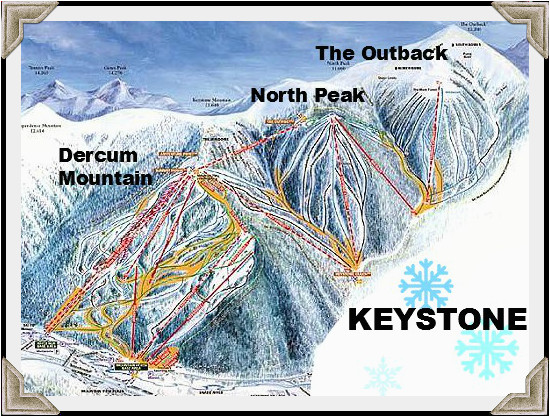This image depicts an artistic rendering, likely a ski map, of Keystone Mountain framed with protective corner cardboards. The frame is marked by a thick black line and the map is a rectangular shape, slightly longer along the top and bottom. The upper portion of the map features a blue sky with white accents, while the main area highlights intricately sketched mountain peaks, primarily moving diagonally from the lower left to the upper right.

Three prominently labeled mountains can be seen: "Durkheim Mountain" on the left-middle, "North Peak" towards the top center, and "The Outback" in the upper right corner. The map features curved, sketch-style lines representing the mountain ranges, interspersed with trails marked in yellow, green, and red. Smaller, less legible text appears to label additional peaks possibly with their heights. 

At the bottom right section, which is a solid white color, "Keystone" is written in large bold all-cap letters accompanied by two blue snowflake icons. The entire scene showcases a blend of various colors including shades of blue, black, white, yellow, orange, green, red, pink, and purple. The overall composition centers on the mountain ranges, creating an impression of a detailed and dynamic ski map or painting.